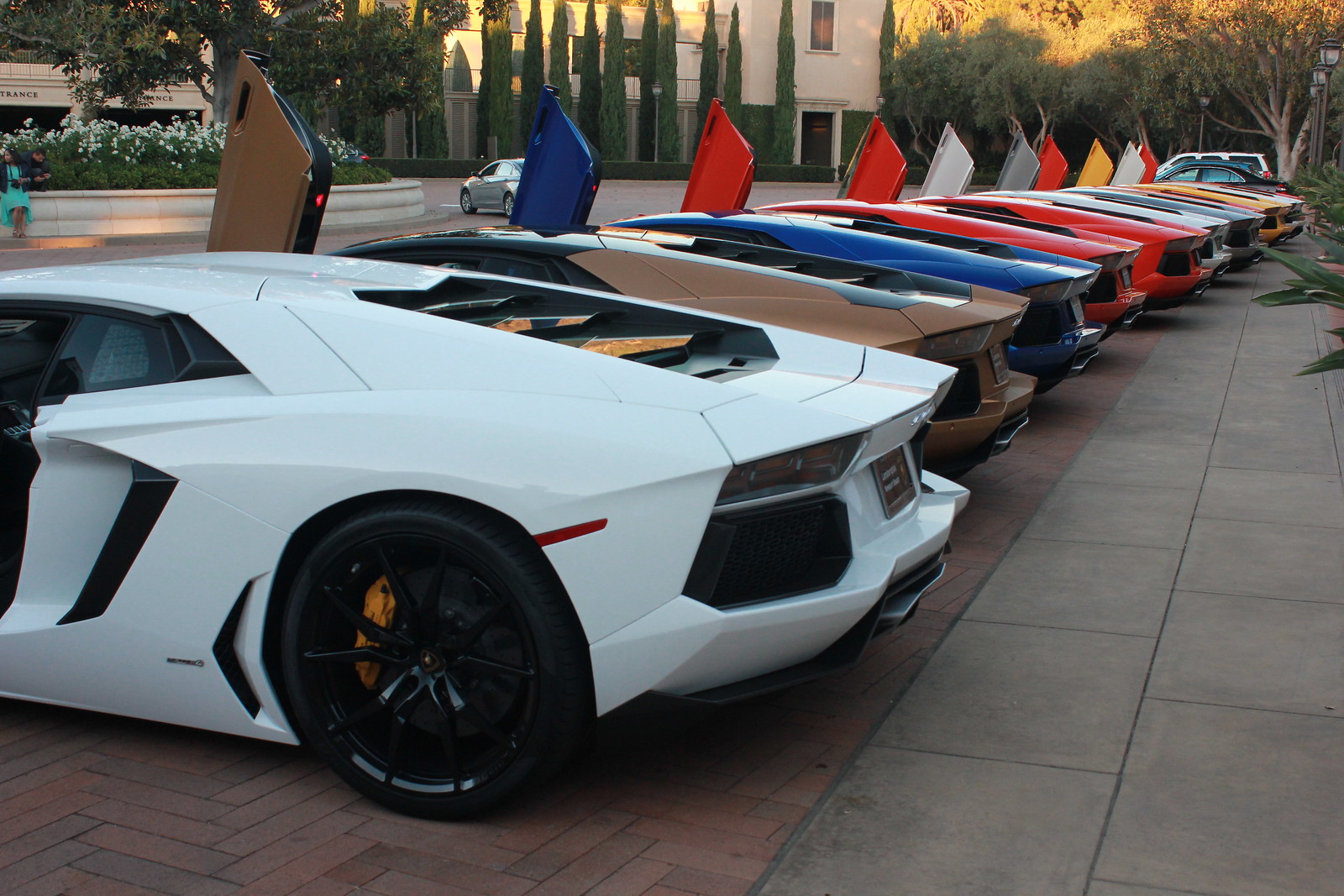In this outdoor photograph taken at a car show or meet-up, a striking row of nearly identical Lamborghinis is featured prominently. All the cars have their scissor doors open, extending upward and emphasizing their sleek, aerodynamic design. The cars, which are parked on a red-patterned brick pavement, include various colors: white, gold, navy blue, multiple reds, yellows, and silver. In the foreground, the white Lamborghini stands out. The background showcases a tree line with lush, deciduous trees and a cream-colored building adorned with tall green bushes. Adjacent to the cars is a circular raised planter, surrounded by tan stone, filled with white flowers and more greenery. Additionally, the pavement extends to the right-hand side with square gray tiles, enhancing the organized yet vibrant setting of this high-end automobile display.